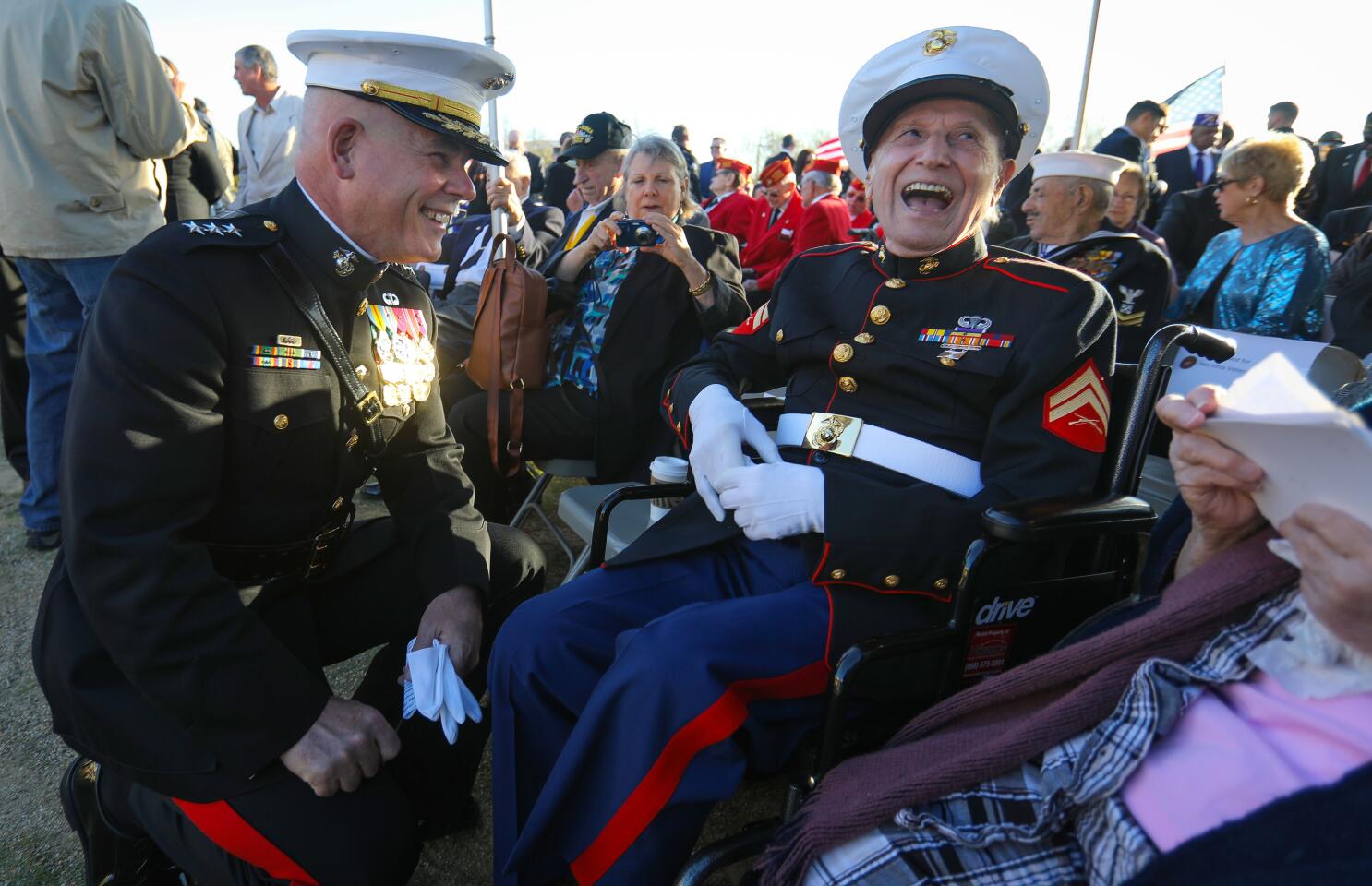In the image, an elderly man in a black wheelchair is prominently featured, his laughter captured in a toothy grin with his mouth wide open. He is dressed in an immaculate military uniform: a dark navy long-sleeve jacket adorned with gold buttons, colorful medals on his chest, and red pointed badges on his shoulders. He wears a white belt with a gold buckle, white gloves, navy pants with a red stripe, and a distinguished white military hat with a black brim and gold embellishments. Beside him, a younger man, similarly attired in an identical military uniform, is kneeling—his white gloves removed and held in his left hand—looking up and smiling at the older man. Both men are bald and the scene is starkly illuminated by a bright, almost washed-out sky. Surrounding them is a crowd of elderly people, likely fellow veterans, some in military attire with white hats, while others include women in dresses and carrying purses. The setting appears to be a veteran's event, given the presence of multiple uniformed individuals and an overall respectful atmosphere. The candid joy and camaraderie between the two men is the heart of the image, embodying a moment of shared history and honor.